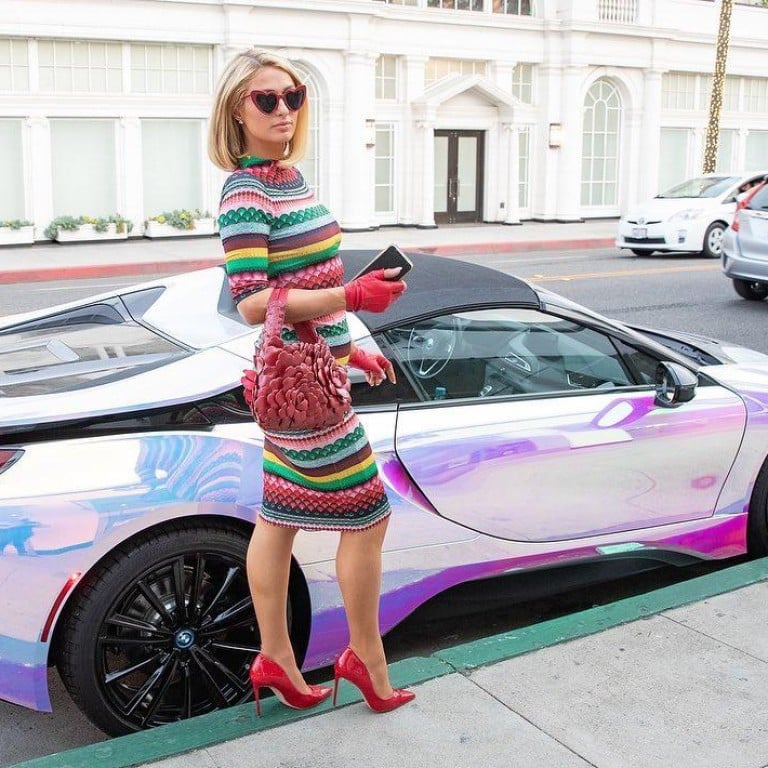This photograph captures Paris Hilton standing on a sidewalk in front of a luxury convertible car with a reflective, holographic silver-pink exterior. Paris, known for her glamorous image, embodies sophistication in a colorful, vertically-striped sweater dress that features shades of blue, green, and a pink that matches her accessories. She dons sleek, shoulder-length blonde hair and heart-shaped sunglasses, adding a touch of playful elegance to her ensemble. Complementing her look are cranberry-colored high heels, a matching pinkish-red purse, and red gloves. Paris holds an iPhone in her right hand, suggesting a candid moment caught on camera. The background reveals a scene of upscale, white buildings suggesting high-end retail stores, further accentuating the affluent vibe of the photograph.